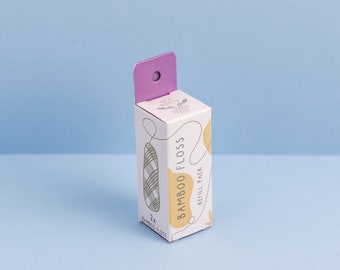The image depicts a small, rectangular box standing upright on a light blue table, with a matching blue wall in the background. The box, intended for hanging on a store hook, features a purple tab at the top with a hole. The main body of the box is predominantly white, accented with green and a yellowish-tan color. On the side, green text clearly reads "Bamboo Floss." Additional, smaller text is present but difficult to decipher. The design on the box includes an illustration resembling a skein of yarn, rendered in gray and white tones, possibly depicting the bamboo floss product contained inside. The overall presentation suggests an environmentally friendly product.